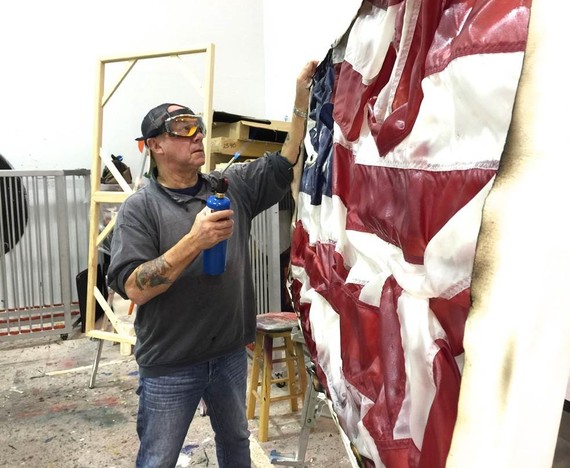The image showcases a Caucasian man standing on dirt outside, marked by a gray or dull-colored sky or wall in the background. He is seen wearing safety glasses and a backwards baseball cap, dressed in a gray long-sleeved shirt rolled up to his elbows with a black undershirt and blue jeans. One hand grips a lit blowtorch attached to a can of butane, while the other holds the corner of a large piece of cloth that resembles the American flag, adorned with red, white, and blue colors and a visible star in the blue field. The cloth appears to be either made of tarp or pinned to a wooden frame or board and shows burn marks around its edges. Behind the man is a white-walled building with a gray fence and a nearby stool.